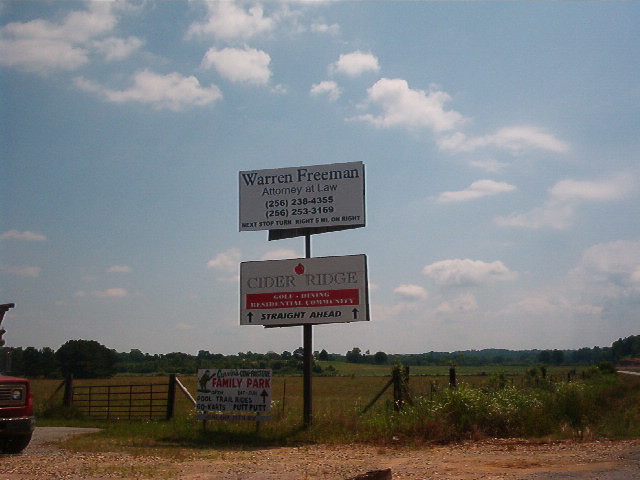In a serene rural setting, three distinct signs prominently adorn a sturdy wooden fence typically used for cattle. The first sign reads, "Warren Freeman, Attorney at Law," accompanied by two contact phone numbers, providing crucial information for legal assistance. Just below it, a sign labeled "Cider Ridge" adds a touch of pastoral charm, hinting at a nearby location or establishment. Attached to the fence as well, a third sign declares "Family Park," inviting visitors to a community gathering place. The backdrop reveals a vast expanse of flatland, interspersed with clusters of trees, all under a brilliant blue sky dotted with fluffy white clouds. In the foreground, lush green vegetation frames the fence, blending seamlessly into the rural landscape. A dirt road, partially visible at the bottom of the image and seemingly photographed from a vehicle, leads the viewer's eye toward the signs, emphasizing the rustic and tranquil nature of the scene.